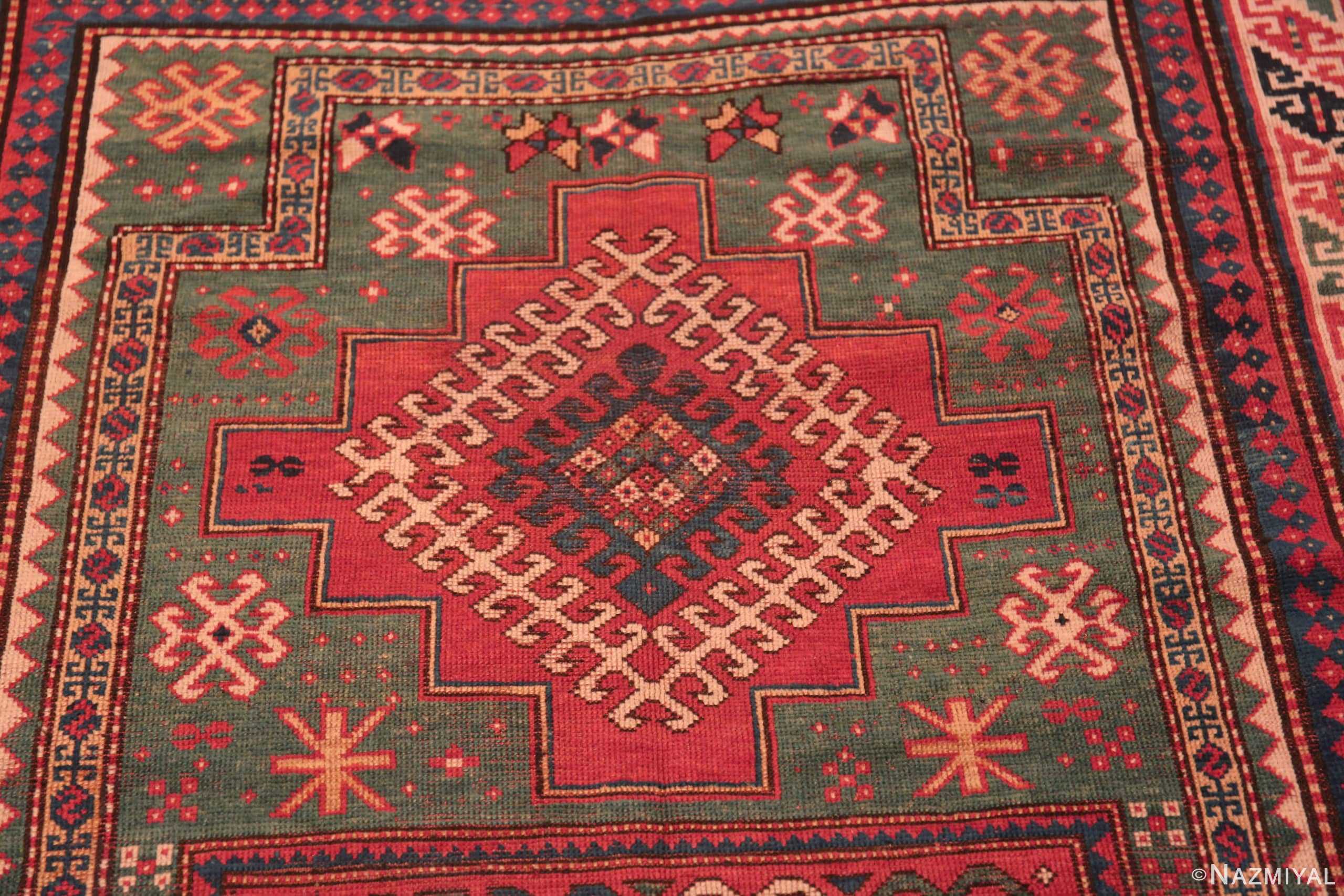The photograph captures a section of a Persian-style rug positioned centrally within the frame. The rug boasts an intricate geometric design dominated by a central diamond motif. This diamond, resembling a rotated square, features a rich red interior bordered by staggered, staircase-like edges. Surrounding the central diamond is a pattern that mimics a star shape, adding complexity to the design. The rug exhibits an array of colors, including greenish-gray, red, yellow, black, and blue, with significant areas of brown and red that highlight the traditional elegance of the piece. The borders of the rug are especially detailed, showcasing a series of green and white triangles, along with a thin black line that encases a blue and red diamond pattern. The outer designs include bands of colors and multiple geometric patterns, creating a visually intricate and appealing appearance that is indicative of handcrafted artistry.